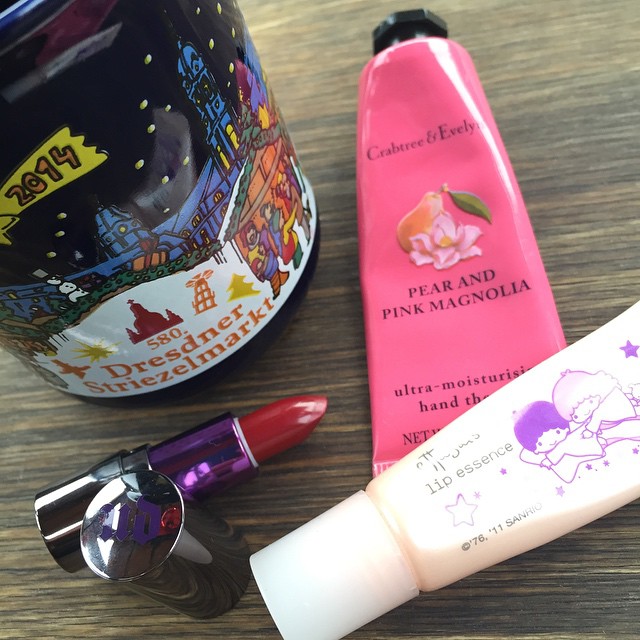In this square photograph, beauty products are arranged on a wooden table with a mix of light and dark brown hues and textured detail. The most prominent item is a pink tube with a black cap featuring an illustration of a pear and pink flower, labeled "Pear and Pink Magnolia Ultra Moisturizing Hand Lotion," though the text is partly cut off. Beneath it lies a white tube tinged with pink, named "Lip Essence," adorned with a purple line drawing of two cartoon characters, one with purple hair and one with white hair, surrounded by stars. Positioned to the left is an open tube of strikingly red lipstick, the lipstick itself fully extended. This lipstick has a silver cap and base, with a purple inner tube. Standing out as well is a jar, labeled "Dresdner Stiesel Mark," showcasing a festive Christmas scene with buildings in snow and the year "2014" written in orange on a yellow background.